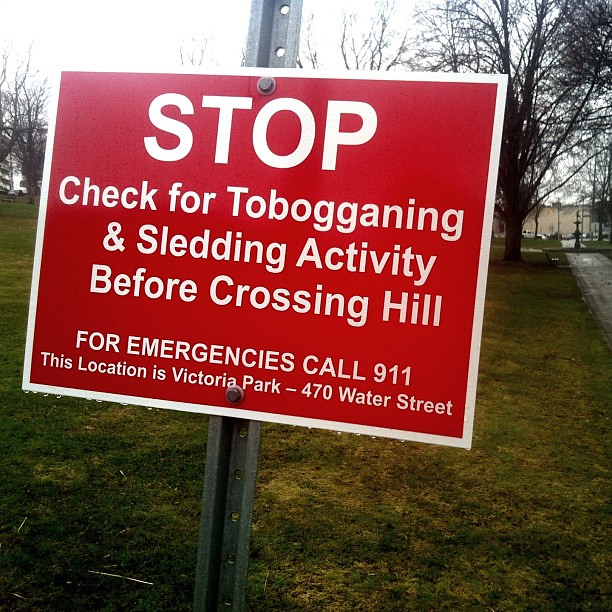The image captures an outdoor scene during a slightly overcast day, likely in early spring or late autumn given the leafless trees and the grass transitioning between green and yellow. Dominating the center of the frame, a metallic gray signpost supports a red sign with a white border and white text. The sign reads: "Stop. Check for tobogganing and sledding activity before crossing hill. For emergencies, call 9-1-1. This location is Victoria Park, 470 Water Street." The foreground features a grassy area with patches of green and yellow, indicating recent seasonal change. To the right, a rain-soaked walkway is visible, and further beyond, a smattering of bare trees outlines the horizon. The sky above is a muted white-gray, completing the serene yet slightly gloomy atmosphere of this public park.